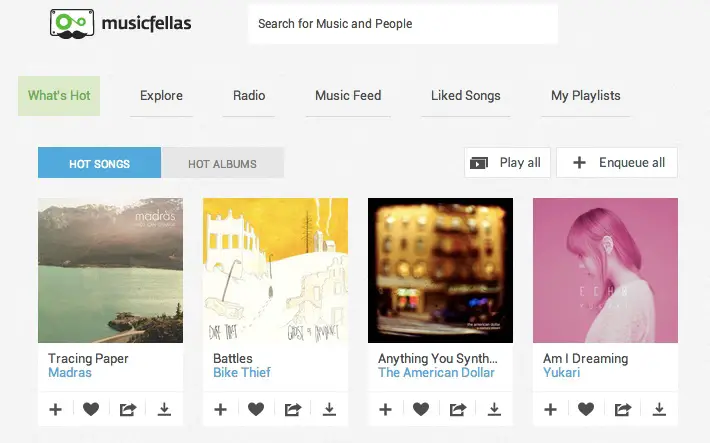In this image set against a solid white background, the upper left corner features a screenshot with the bold black text "Music Fellas" accompanied by a distinct logo to the left. Adjacent to this, on the right, is a search bar with the placeholder text indicating the ability to "Search for music and people." The navigation menu spans from left to right, beginning with "What's Hot?" in a light green box. Following that, in black text, are the options: "Explore," "Radio," "Music Feed," "Liked Songs," and "My Playlist." In the lower left corner, there is a blue action button labeled "Hot Songs" in white text. To its right, "Hot Albums" is presented inside a gray box. Below this are four album covers with their corresponding titles and artists listed. The first album is "Tracing Paper" by Madras, followed by "Battles" by Bike Thief. Next is "Anything You" by The American Dollar, and lastly "Am I Dreaming" by Yukari.